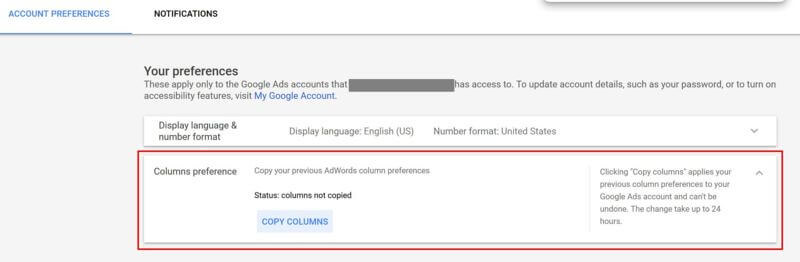This color photograph appears to showcase a segment of a website or web page, possibly related to Google Ads account settings. The layout includes various sections and text that describe different account preferences and options.

In the upper left corner, there is a header with "Account Preferences" written in blue text on a white background. A blue underline extends from this header over a grey line that runs horizontally across the page, separating different sections.

To the right of the header, "Notifications" is displayed in black text. At the very top, a thicker grey line indicates the boundary of another section.

Beneath these sections is a grey background featuring the heading "Your Preferences" in black text. This is followed by a description stating, "These apply only in the Google Ads account." Further down, there is a blocked-out section of text, presumably containing sensitive information.

Continuing on, the page explains, "To update account details such as your password or to turn on accessibility features, visit My Google Account." The phrase "My Google Account" is highlighted in blue text, indicating it is a clickable link.

Under this, there is a light-colored rectangular area featuring black text, which states "Display Language and Number Format." Below this section is another block of text surrounded by a red rectangle, indicating custom preferences.

At the very bottom, a blue button labeled "Copy Columns" stands out. To the right side of the image, there is additional black text that is unreadable due to its small size.